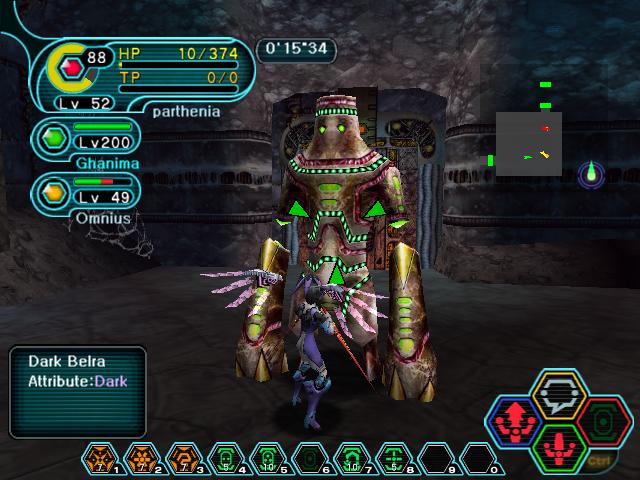The image depicts a character from a video game, showcasing a detailed and unique design. The character has a square head with striking green eyes and green accents surrounding the head, which is notably flat. The figure lacks a neck and features a coloration of green and maroon around the upper chest area. The character's arms are disproportionately large, ending in club-like extensions. The thin body is composed of various lines and geometric shapes, adding to its distinctive appearance.

In the foreground, to the side of the main character, there is a small purple figure that appears to be wearing high heels, possibly indicating it is a female character. The main character seems to be navigating a dungeon-like environment. There is text in the upper left-hand corner of the image that reads "Dark Belcher" with the attribute labeled as "Dark." Additionally, there are colored boxes displayed along the bottom and in the lower right corner of the image, likely representing different game elements or stats.